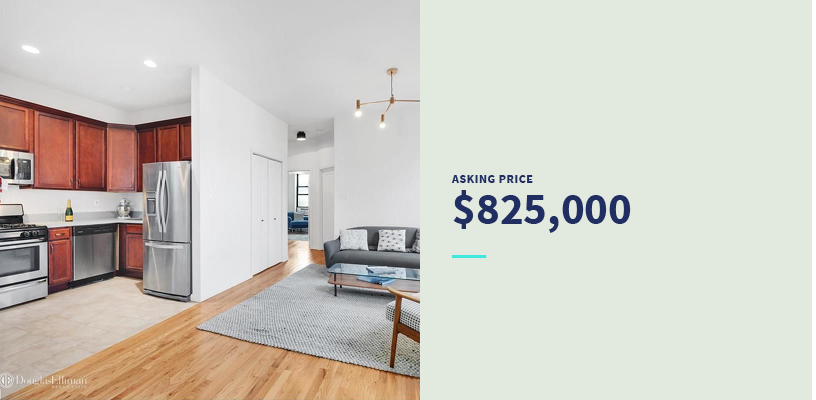This image is a screenshot of an advertisement for what appears to be a residential property, either an apartment or a house. The screenshot is divided into two distinct sections. On the left side is an interior photograph showcasing a portion of the home's kitchen and living room. The kitchen features a silver refrigerator and brown wooden cabinets, set against beige-colored tile flooring. A small wall partially separates the kitchen from the living room area. In the living room, there is a gray couch adorned with two white pillows, a gray carpet, and beige or brownish wooden floors. The walls throughout the home are painted white, contributing to a clean, bright appearance. On the right side of the screenshot, text prominently displays the asking price of the property, listed at $825,000. This suggests that the advertisement is likely part of a real estate listing, either from a realtor or a real estate website.